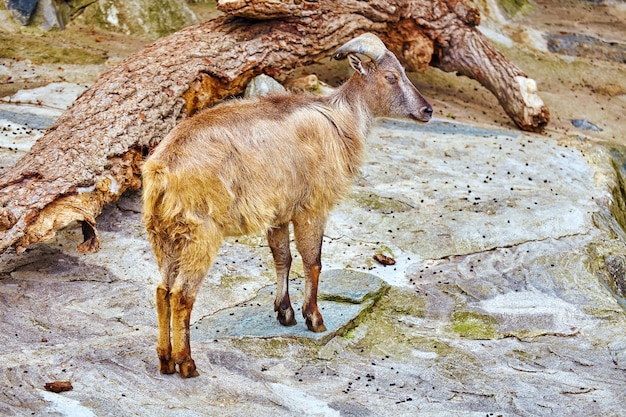The photograph depicts a four-legged animal standing on a rocky formation that is relatively flat but distinctly made of rock, possibly within a zoo setting, though the environment suggests a natural habitat. The animal, identified as a goat, is positioned beside a large, misshapen tree trunk that lies parallel to the ground, likely a fallen branch that the goat may have nibbled on as goats are known to chew on various objects. The surrounding area consists of greenish-brown dirt, indicating flat land around this stone hill and tree trunk. Scattered across the rocky surface, there are numerous small black pellets, likely goat droppings, hinting that this is a frequented spot for the goat. The goat itself is of medium size, covered in shaggy, brownish-tan fur. It features short, curved horns on either side of its head and has pointed, backward-curling ears. The animal stands very still, with its back legs together, surveying its surroundings.